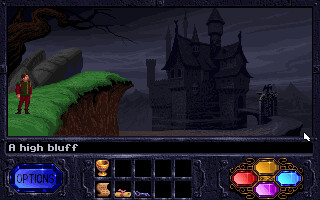In this screen capture from a mobile RPG game, the primary focus is a hauntingly detailed, old-school Bavarian mansion, reminiscent of the Beast's castle from "Beauty and the Beast." The mansion, along with its surroundings, is enveloped in varying shades of gray, including its stone facade, the overcast sky, the cobblestone road, and the wrought-iron gate that guards the property. This monochromatic setting exudes an eerie, foreboding atmosphere. 

In stark contrast, off to the left, a character stands on a grassy cliff, adding a splash of color to the scene. Dressed in a mix of red and green attire, the character's brown hair complements the vibrant yet rugged environment, featuring a gnarly tree and jagged rocks. The cliff sharply drops off to the grayscale road below, adding a dramatic element to the composition.